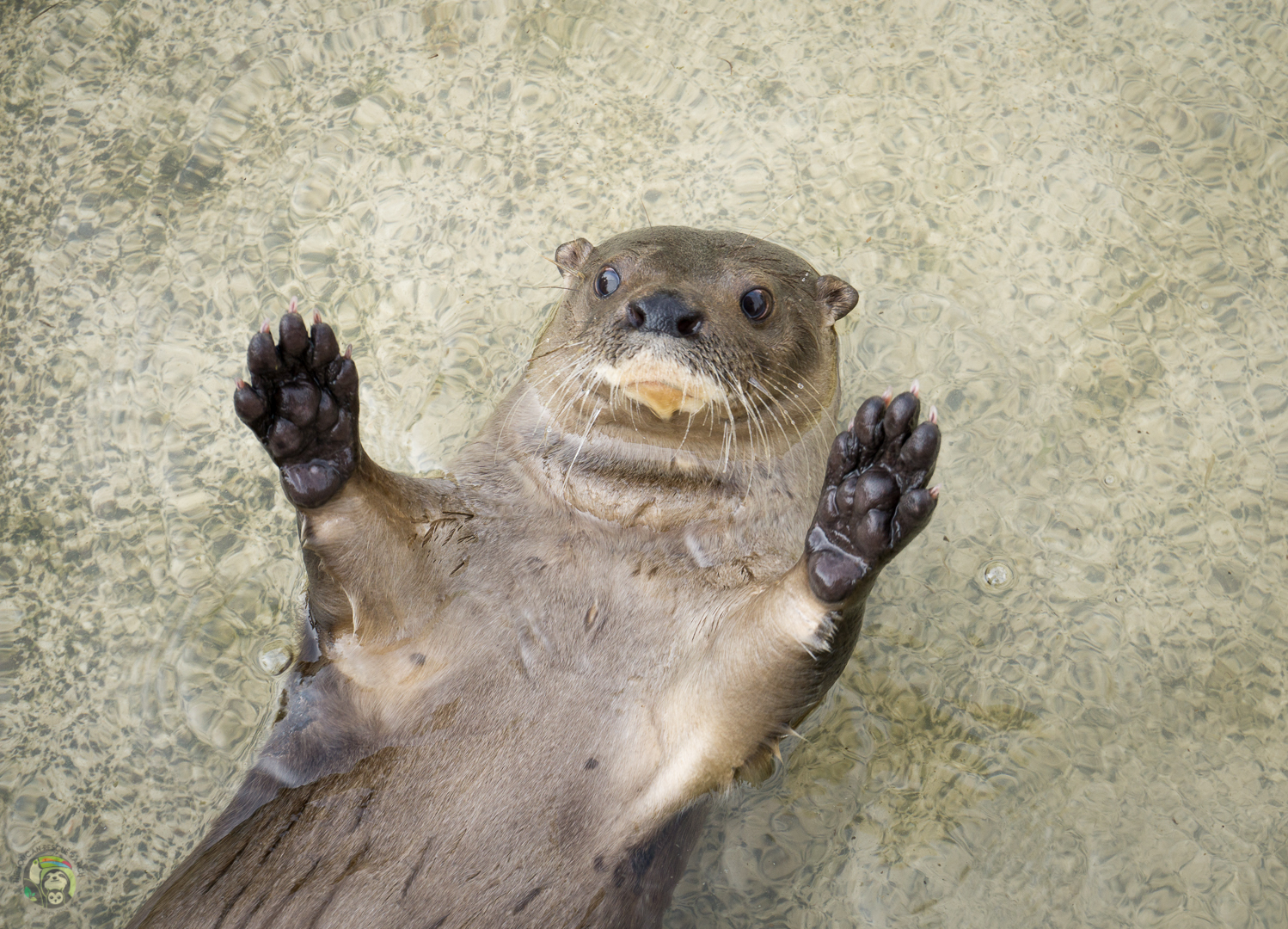The photograph depicts an otter floating on its back in a body of clear water, with the image taken from above. The otter's face, belly, and front paws are visible, with its body extending towards the lower left side of the frame. The otter's fur is a blend of various shades of brown, with black splotches on its tummy and black-colored paws. Its fur appears matted and smooth, suggesting it is wet. The otter has small black eyes, a black nose, and its whiskers seem to have water droplets on them. Its face is blunt with small ears at the corners, and there is a white area around its upper lip. The otter's little palms and five-fingered paws with claws are spread out, and it has something beige or golden in its mouth. The water beneath the otter is very clear, revealing a green base made up of light and dark green pebbles, with some pebbles appearing embedded in a solid substance. Ripples and a small bubble to the right of the otter indicate the presence of water.